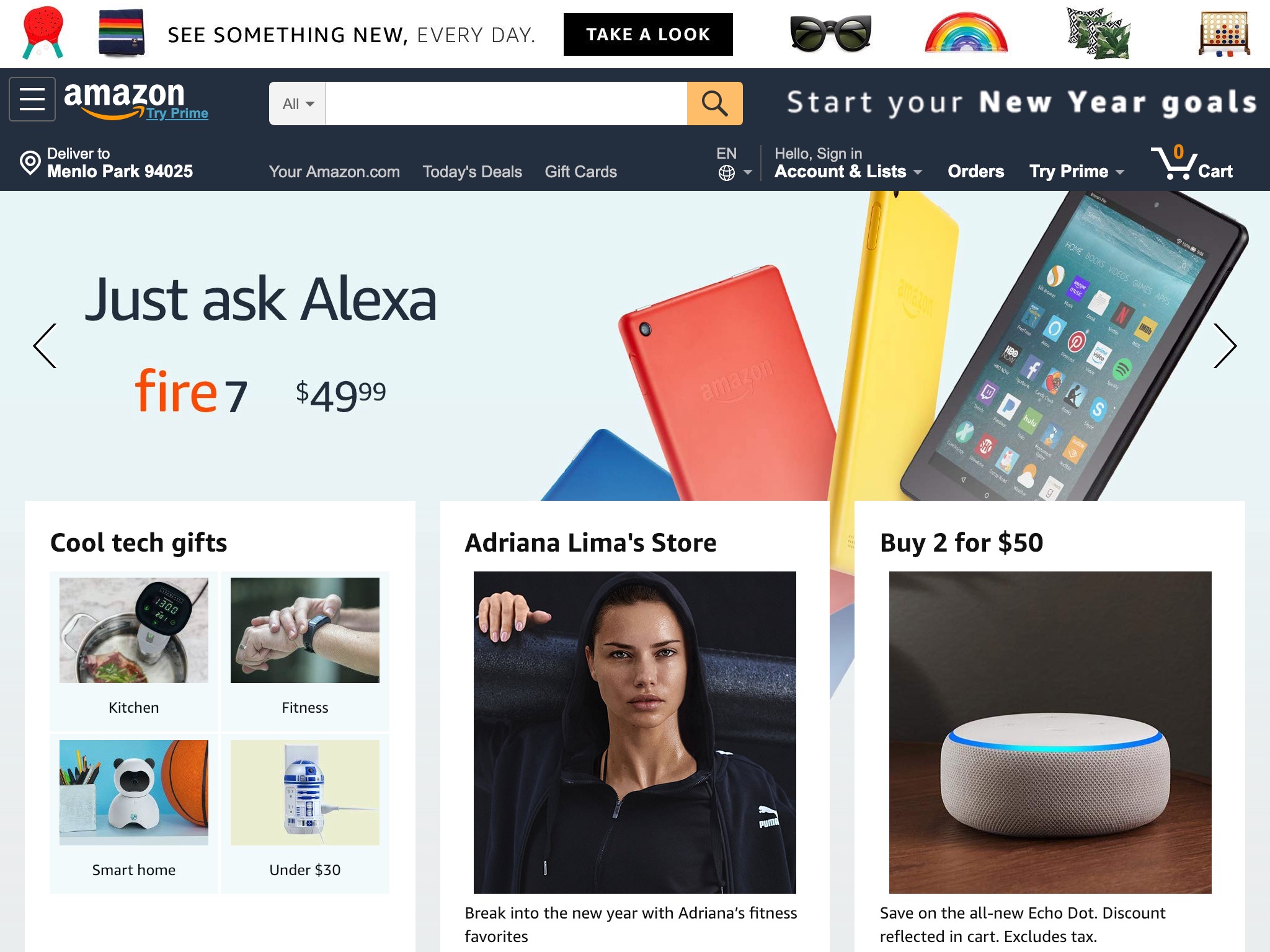This is a detailed caption describing an Amazon webpage:

The top left corner of the Amazon webpage features the word "Amazon" in white font with the iconic gold arrow starting under the letter "a" and pointing towards the letter "z." Adjacent to this, in blue font, are the words "Try Prime." Right next to it is a white search box, and to the right of the search box, there’s a promotional message in white font that says "Start your New Year goals."

Above this section, on the left side outside of the main Amazon area, there are several small graphic elements, including red ping pong paddles with turquoise handles and some other indistinguishable items. Additionally, there's text in black font that says "See something new" followed by "every day" in a lighter font. Beneath this text, in a black horizontal rectangular box with white font, it says "Take a look." Further down, there are icons featuring sunglasses, a rainbow, and some other indistinct graphics.

At the very top of the webpage, it says "Deliver to Menlo Park 94025" in white font on a dark background. In the center to the left, there's a greeting "Hello, Sign in," followed by "Accounts & Lists," "Orders," "Try Prime," and a shopping cart icon with a gold number zero above it and the word "Cart" next to it.

In the main area, a large message at the top reads "Just Ask Alexa" with an illustration below. Following this, in large orange text, it says "Fire 7" priced at "49.99." Below this are images of phone cases in various colors: blue, orange, yellow, and black with the black phone case facing outwards. On the left side, there are four horizontal rectangular buttons with labels and images: "Kitchen" with a meat thermometer, "Fitness" with an image of an arm wearing a fitness tracker, "Smart Home" with a small white character and basketball, and "Under $30" featuring a small robot.

Next to these are two larger vertical rectangular sections. The first one reads "Adriana Lima's Store" in black font and features a picture of Adriana Lima wearing dark clothing and holding a foam roller behind her back. Below her image, there's text that says "Break into the New Year with Adriana's fitness favorites." The section next to it highlights a promotion "Buy 2 for $50" showing an image of a white Echo Dot with a turquoise rim. Below the image, it says "Save on the all-new Echo Dot. Discount reflected in cart, excludes tax."

This detailed caption encapsulates various elements and sections of the Amazon webpage, giving a comprehensive description of its layout and content.